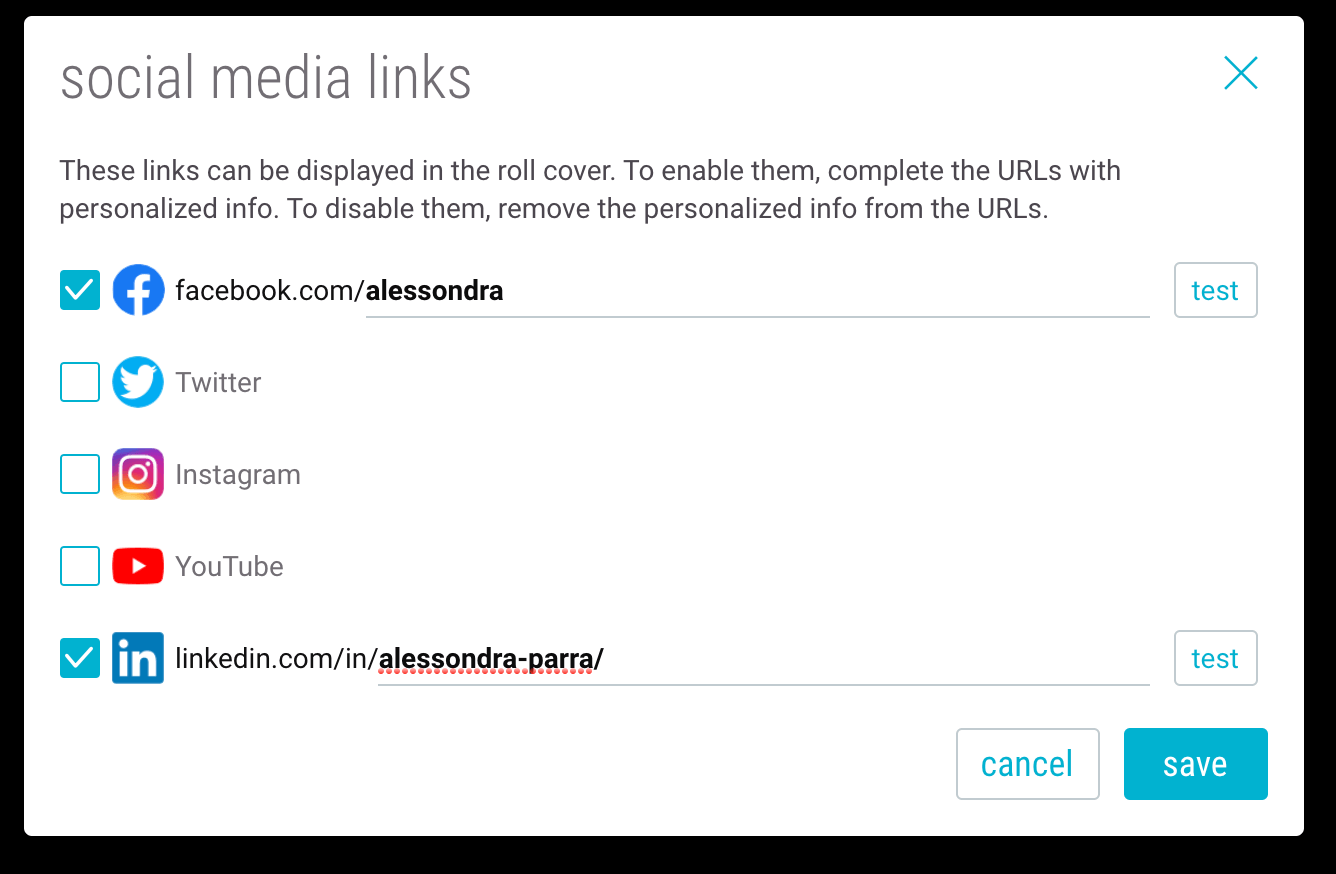This image captures a web page section dedicated to managing social media links. At the top-left, there are social media icons indicating the section's purpose, while the top-right corner features a closeout 'X' button. The main text instructs users on how to enable or disable these links: "These links can be displayed on rollover. To enable them, complete the URLs with personalized info. To disable them, remove the personalized info from the URLs."

Below this instruction, there are several social media links listed with checkboxes next to each. The first link, which is checked, shows the Facebook logo followed by "facebook.com/Alessandra," accompanied by a test button on the far right. The second link, which is unchecked, displays the Twitter logo and the text "Twitter." The third entry, also unchecked, features the Instagram logo and the word "Instagram." The fourth unchecked link has the YouTube logo and "YouTube." The last link is checked and includes the LinkedIn logo followed by "linkedin.com/in/alessandra-para/," with a corresponding test button on the far right.

At the bottom right of the section, there are "Cancel" and "Save" buttons for applying changes. This web page section effectively allows users to manage their social media visibility by toggling checkboxes and editing URLs.